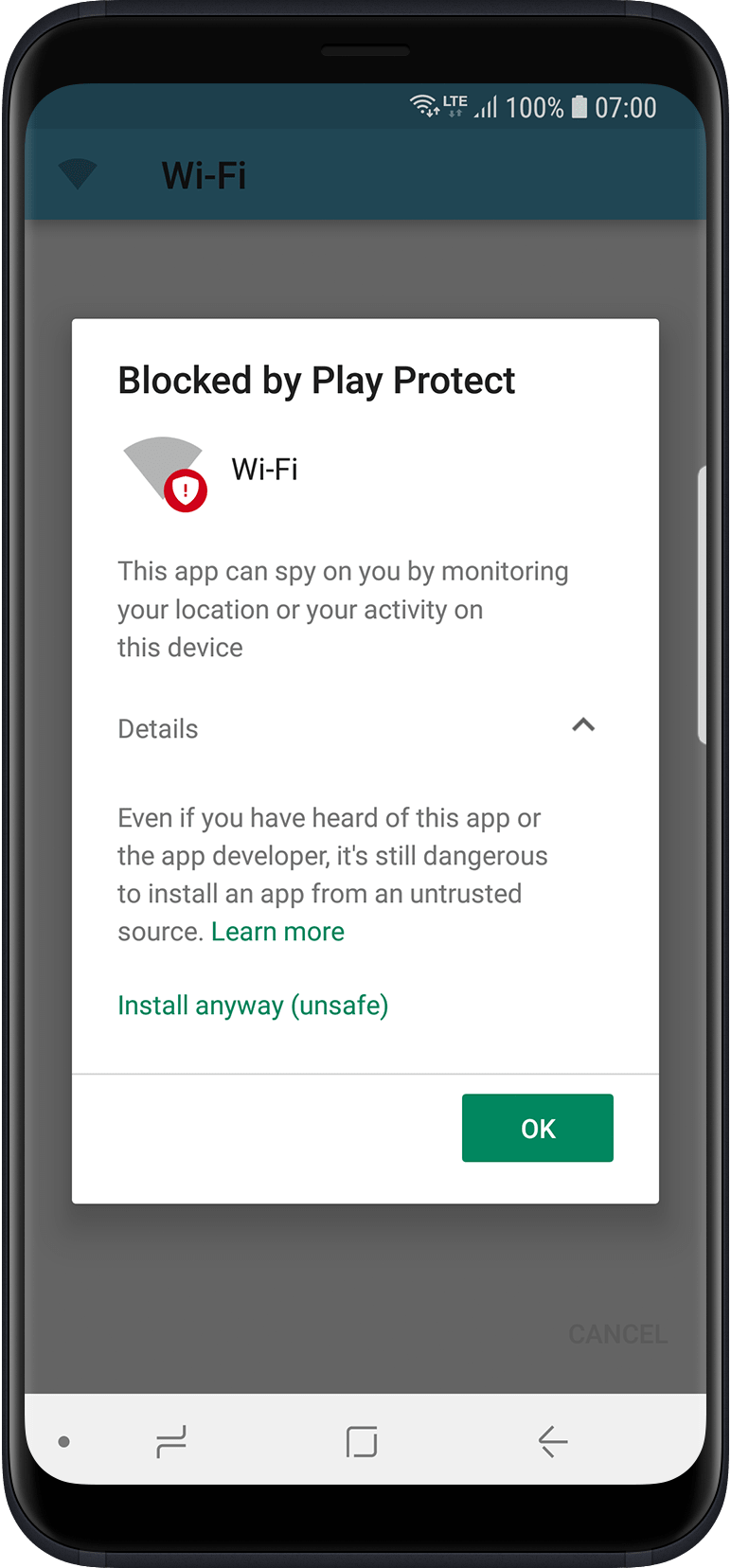The image depicts a smartphone screen with several details visible. At the top of the screen, the status bar shows the Wi-Fi symbol and the network signal indicator, accompanied by the text "_LTE_" and a 100% battery level notation. The time displayed on the device is 7 o'clock. The screen is dominated by a security warning from Google Play Protect, alerting the user about a potentially harmful app. The warning message indicates that the app may spy on the user's location or activities on the device, cautioning that even if the user is familiar with the app or its developer, it is dangerous to install apps from untrusted sources. The message includes green text with the option to "Learn more" about these risks. Below this, there are two buttons: one labeled "Details" and another labeled "Install anyway" within parentheses. At the bottom right corner, there is an "OK" button to acknowledge the warning.